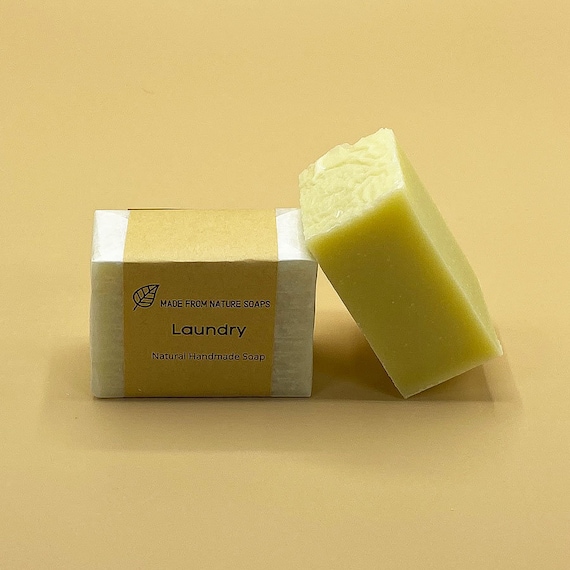This photograph features a detailed scene centering on a yellow rectangular bar of soap resting on a yellow surface. The bar of soap is unwrapped and prominently displays its natural, handmade composition. Adjacent to it, a similar rectangular object, wrapped in white paper with a yellow label, leans against it. The label on the wrapped soap includes several elements: at the top, it reads "Made from Nature Soaps" accompanied by an illustration of a leaf. Below this, the word "Laundry" is inscribed in black text, followed by "Natural Handmade Soap." The yellow hue of the soap suggests it might be made from ingredients like lemon or banana. The overall setting is minimalistic, with a focus on the organic and handmade qualities of the soap.